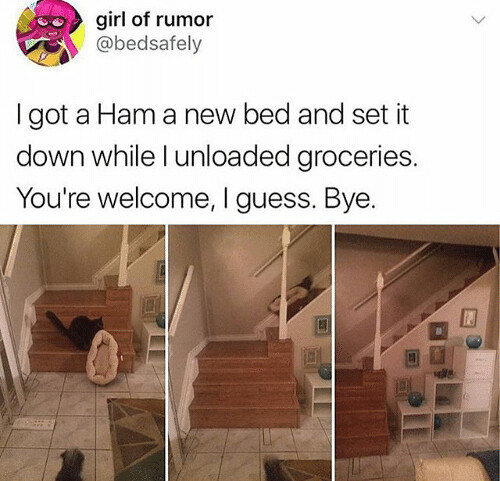This image is a humorous Instagram post by user @girlofrumor, captured from a tweet. The caption reads: "I got a ham a new bed and set it down while I unloaded groceries. You're welcome, I guess. Bye." The post consists of three sequential images featuring a comical scenario. The first image shows a black cat at the bottom of a staircase, gripping a pet bed in its mouth. The beige tile floor, brown stairs with white railings, and a beige wall can be seen in the background. The second image captures the cat mid-action, beginning to ascend the stairs with the bed. The third image shows the stairs now devoid of the cat, indicating it successfully carried the bed upstairs, leaving only the frames, shelving, and an area rug in various shades of brown visible. The series of images humorously documents the cat's determined journey.